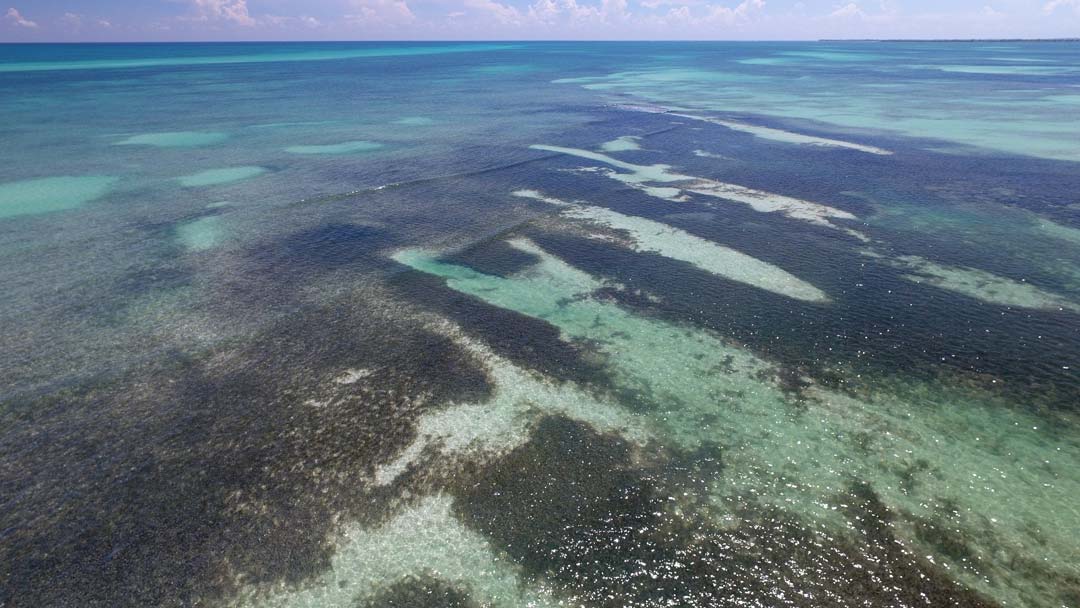This aerial view of the ocean captures a striking scene where crystal-clear waters meet various shades of blue and green. The background reveals a gradient of turquoise blue deepening to dark blue, likely indicating different depths or sections of a coral reef. Predominantly clear, the water allows visibility to underwater vegetation, including patches of seaweed and possible reef areas, though actual coral is sparse. The submerged beach or island areas are marked by dark green and brown patches, giving a textured, almost dirty appearance to some sections of this expansive, clear ocean. Ripples on the water's surface and small, color-varied puddles accentuate these dark vegetated zones, adding intrigue and complexity. Above, a narrow strip of sky, tinged with clouds of cyan, pink, and white, suggests it's daytime, enhancing the overall brightness of the scene.